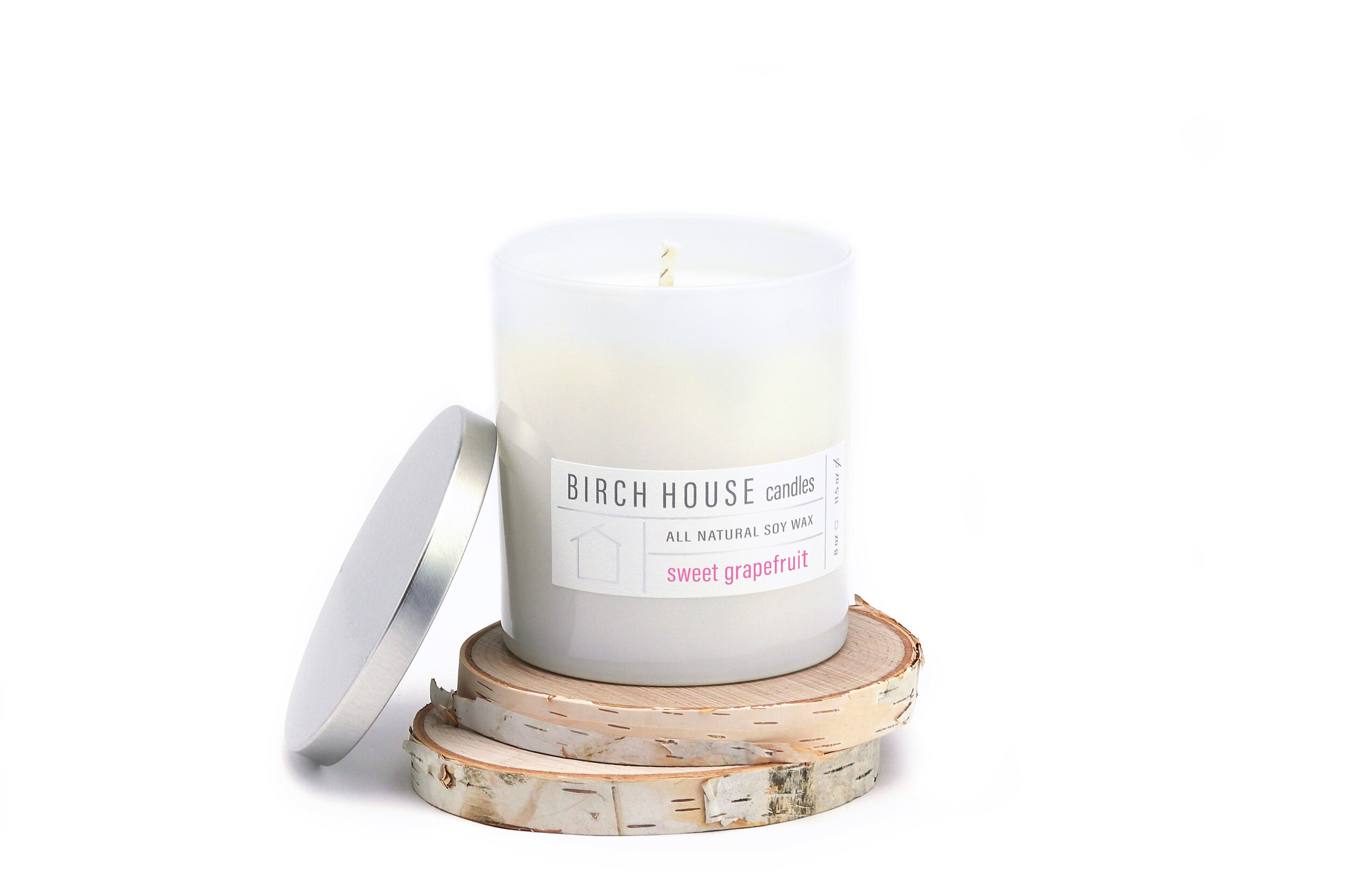In this detailed color photograph, presented in a square format, the central focus is a white jarred soy candle from Birch House Candles, prominently displayed on a transparent, white background that emphasizes a clean, modern aesthetic. The candle is housed in a short, round, whitish glass container with a white wax candle inside, featuring a slightly protruding wick topped with subtle black specks, indicative of its new condition. Leaning against the left side of the candle holder is a sleek, silver screw-on lid. The candle sits atop two stacked circular coasters made from birch wood, with a contrasting texture of bark on the edges and light wood on the inner surfaces. A white label on the candle's front prominently displays in black text, "Birch House Candles" followed by "All Natural Soy Wax." The product scent, "Sweet Grapefruit," is highlighted beneath in a rich purple or pink hue. Adjacent to the text is a simple line art illustration of a house. The overall setup suggests a product or catalog display photography, emphasizing realism and representational photography.